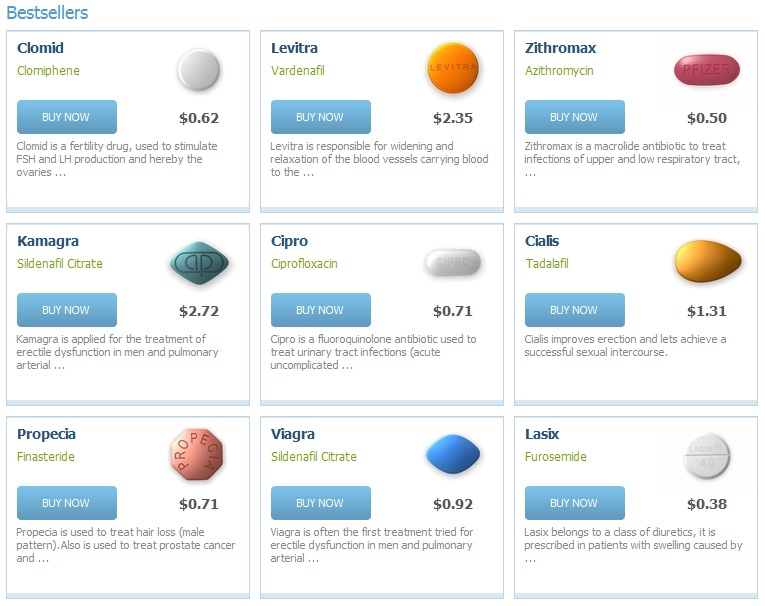This image showcases the top 9 best-selling medicinal tablets, each neatly presented in individual boxes on a clean white background. The boxes feature light sky blue outlines and include an image of the pill, its price, a "Buy Now" button in darker blue, and a brief description.

1. **Clomid** - A white circular pill.
2. **Levitra** - An orange circular pill.
3. **Zithromax** - A burgundy red pill oriented horizontally.
4. **Kamagra** - A diamond-shaped pill.
5. **Cipro** - A white tablet pill.
6. **Cialis** - A gold pill resembling a sunflower seed.
7. **Propecia** - An octagonal tablet.
8. **Viagra** - An oval-shaped blue pill.
9. **Lasix** - A white circular pill.

The prices of these medications range from $0.30 to $2.72.